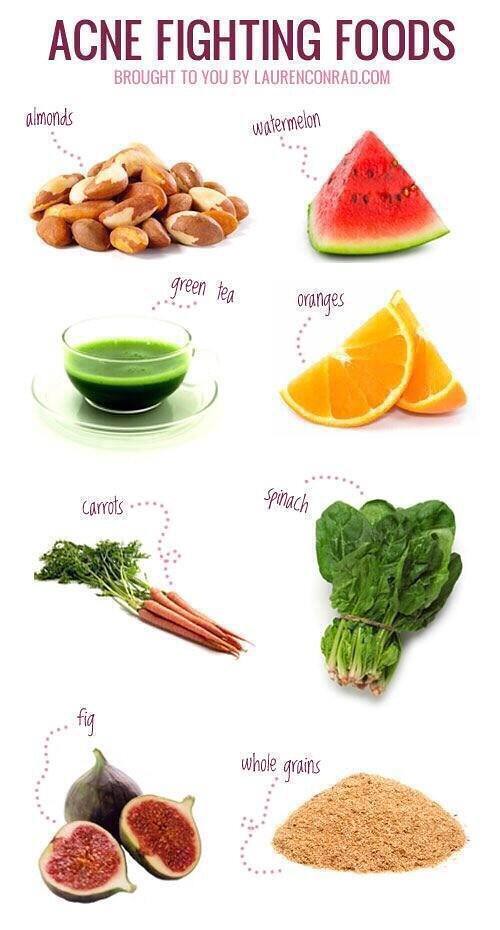The image features a clean white background with the title "ACNE FIGHTING FOODS" prominently displayed in large, uppercase purple letters at the top. Below the title, in a smaller font, it reads "brought to you by laurenconrad.com." The centerpiece of the image is a colorful array of labeled photographs of various foods, each known for their potential benefits in combating acne. 

From left to right, the foods displayed include a pile of almonds, a slice of watermelon, a clear cup of green tea on a clear saucer, slices of oranges, a bunch of carrots with their green tops still attached, a bunch of spinach, two figs (one whole and one cut open to show the inside), and a pile of whole grains. Each food item is clearly labeled to avoid any confusion. The bright and detailed images of the food set against the white background offer a clear and appealing visual guide to acne-fighting foods.